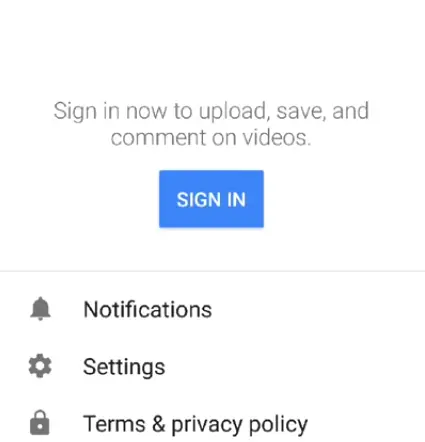The image depicts a mobile screenshot of a sign-in screen with a minimalist design and a predominantly white background. At the center of the screen is a periwinkle blue button with sharp edges, prominently displaying the words "SIGN IN" in bold, white, capital letters. Above this button, there is a gray, two-row text segment: the first row reads "Sign in now to upload, save," and the second row continues with "comment on videos." 

Below the sign-in button, a thin, gray, horizontal line stretches across the width of the screen. Beneath this line, the word "Notifications" appears, accompanied by a small gray bell icon to its left. Following this, the word "Settings" is displayed, paired with a small gear icon also in gray, featuring six teeth and positioned to the left.

At the bottom of the screen, the text "Terms and privacy policy" is shown, with a small lock icon to its left, emphasizing the security aspect of these terms.